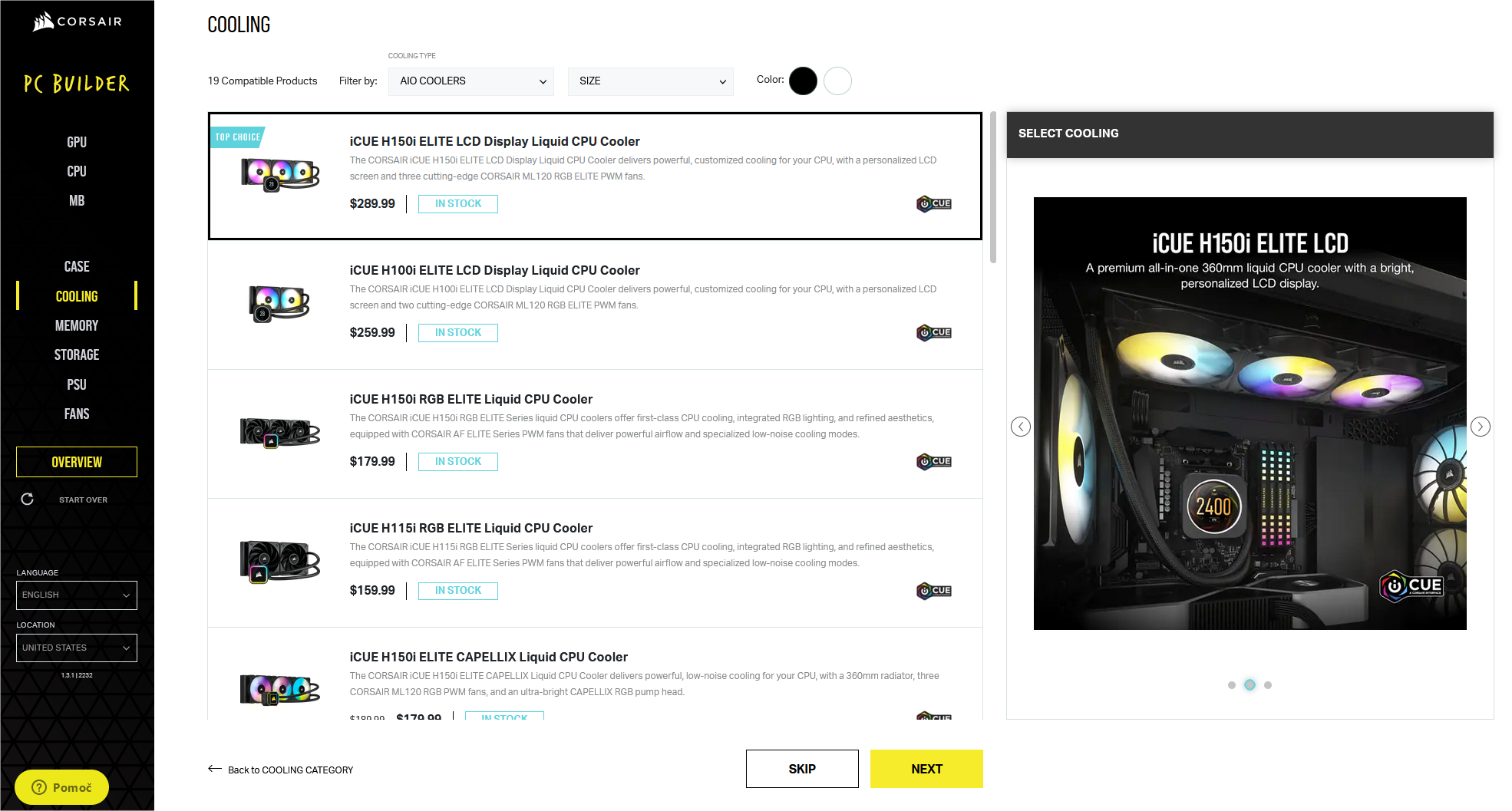This image is a detailed screenshot from a website, showcasing a page dedicated to PC component customization. 

On the left side of the screenshot, there is a black sidebar running from top to bottom. At the very top of this sidebar, "Corsair" is written in thin, white, capital letters, accompanied by a white icon depicting three computer towers, denoting the PC manufacturer, Corsair. Below this logo, in a yellow font reminiscent of handwritten block letters, it reads "PC Builder." The sidebar continues with a vertical list of components including GPU, CPU, and MB. A small space separates this list from the next section, which includes Case, Cooling (highlighted in yellow to indicate the current page), Memory, Storage, PSU, Fans, and Overview in yellow.

The main section of the page, with a white background, features a black headline at the top, labeled "Cooling." Below the headline, multiple CPU coolers are listed, each accompanied by a small photo of the product. These coolers are rectangular units with three round, multicolor, iridescent disks.

At the top of the product listings, the highlighted item is marked with a small blue banner on the left, reading "Top Choice." This top choice product is the ICUE-H150i Elite LCD Display Liquid CPU Cooler, priced at $289.00, though another figure, $299.99, is also noted. Each subsequent product follows the same listing format.

On the far right side of the page, there is a larger photo of one of the cooling units. The unit is black and prominently features the three iridescent disks, indicative of the product’s design and functionality.